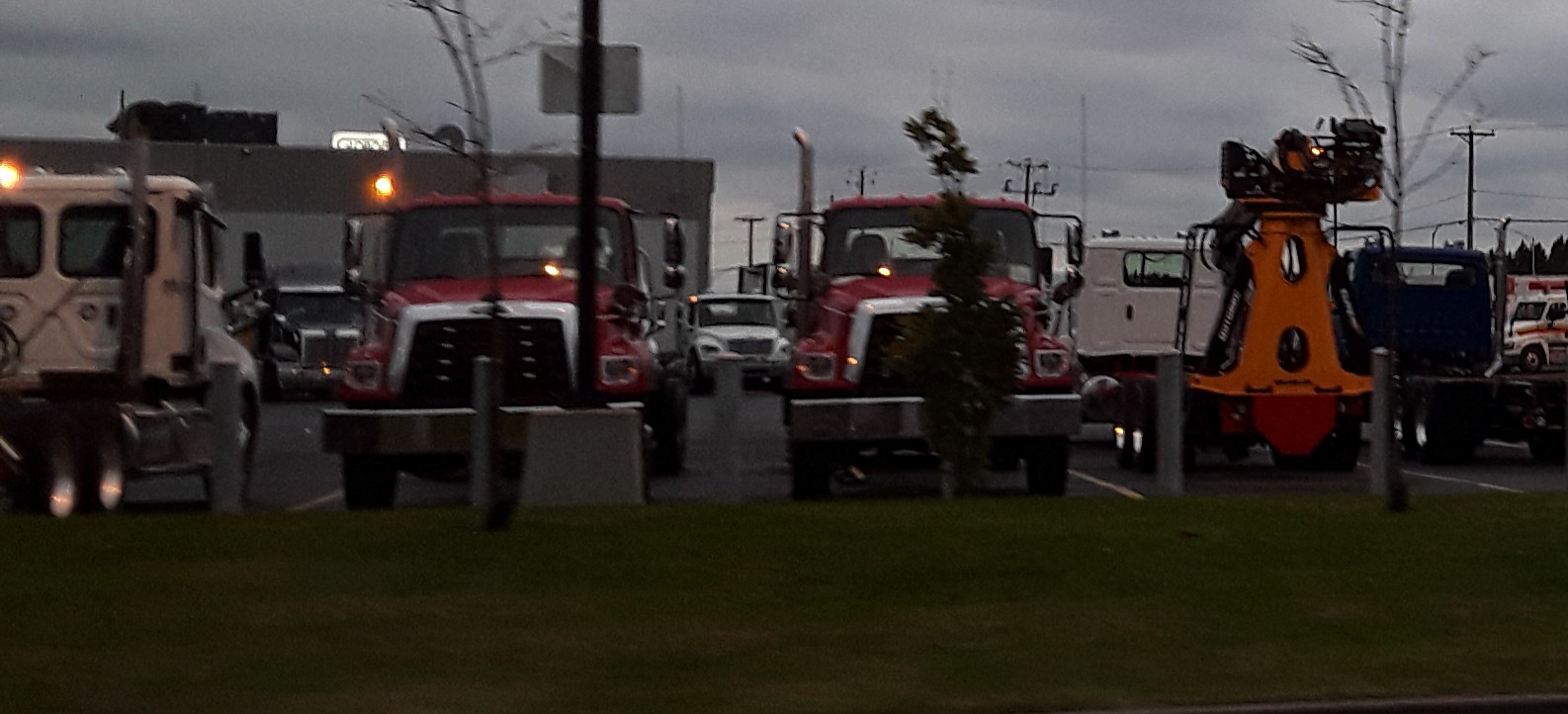This horizontal, rectangular photograph captures the twilight atmosphere of a truck stop or parking lot as night falls. In the foreground, three semi-tractor trailer trucks are prominently parked on a dark charcoal gray surface. On the left, a white semi-cab stands in profile, showcasing a silver smokestack on its side. Centered in the image are two nearly identical red trucks, distinguished by their white-edged grills and similarly placed silver smokestacks.

To the far right, a large red, somewhat triangular object, possibly a construction machine or a loader device with visible orange hydraulic cables, adds intrigue. Behind this, various white cars are scattered, oriented in different angles. Further back, a low, one-story building with light-colored walls and a darker roof can be seen, hinting at the facility's purpose. The sky looms dark gray and overcast, filled with heavy clouds, casting an overall shadowy and somewhat blurry ambiance.

A streetlight or security light, partially obstructed and mounted on a concrete pillar, is visible just left of center, casting enough light to make out green grassy areas with small trees at the image's edges. Despite the dark and somewhat poor quality of the photo, the scene effectively conveys the quiet solitude of a truck yard preparing for nightfall.